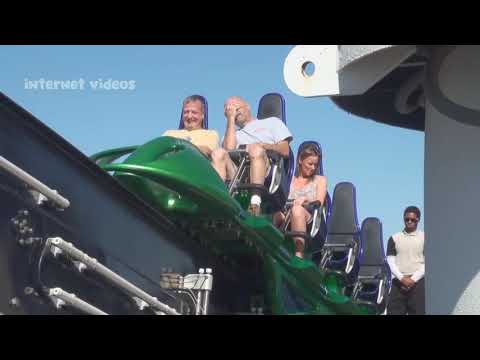The image depicts a grainy, low-quality photo of a green roller coaster in motion, just starting its climb on the track. The track is a contrasting dark, possibly black color, with visible metal mechanical parts at the foundation. The bright blue sky provides a backdrop. 

In the front row of the roller coaster car, there's an older couple showing mixed emotions. On the left, an elderly woman in a yellow t-shirt smiles, while on the right, an elderly man in a white t-shirt appears concerned, covering his face with his hand. Both seem to be in their 70s or 80s. Behind them sits a middle-aged woman, followed by two empty seats. Standing beside these empty seats is a Black man, likely a ride attendant, observing the scene. 

The roller coaster seats are black, matching the track's machinery, and on the top left corner of the image, the phrase "internet videos" is visible in blurry, transparent white text.